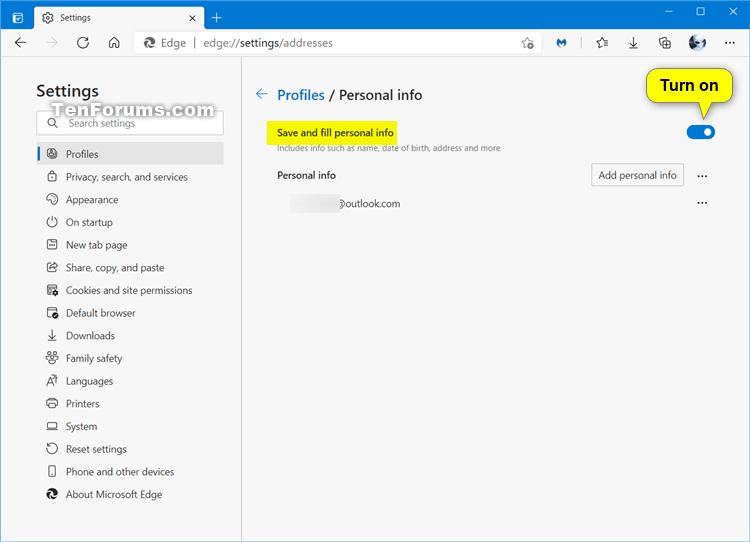This image is a screenshot of the settings page from the 10forums.com website, as evidenced by their watermark located approximately one-eighth to one-sixth of the way down the left-hand side of the page. The watermark consists of white text with a smoky gray backlighting or glow effect. 

The top portion of the page is marked by a blue header containing a white tab labeled "Settings." The rest of the page features a white background adorned with predominantly black text. Notably, there is a blue, clickable word followed by an arrow that provides an option to navigate back.

The browser in use is Microsoft Edge, with the screenshot specifically capturing the "Settings" section of Edge. On the left side of the settings page, there is a vertical menu listing various categories beneath the "Settings" header, accompanied by a white search box at the top of this menu.

The main content area to the right highlights that the "Profiles" category has been selected, and within that, the "Personal info" section is currently open. Within this section, there is a prominent yellow box with black text indicating "Save and fill personal info." Adjacent to this, on the far right of the page, is a yellow speech bubble with the text "Turn on," which is directed at a toggle option to enable this feature.